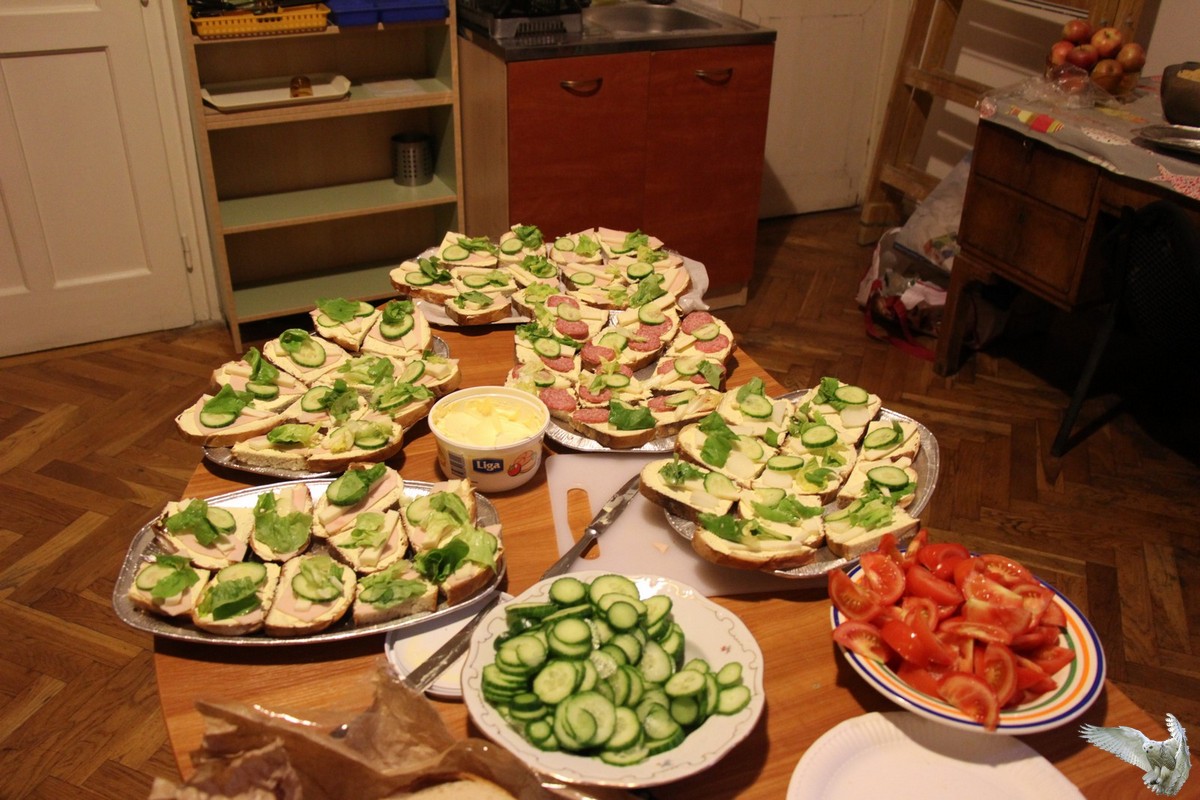This detailed photograph captures a cozy kitchen setting with a focus on a wooden table laden with various ingredients, presumably for assembling sandwiches. Dominating the table are large silver platters, each holding single slices of bread topped with a variety of ingredients including deli meat, lettuce, cucumber, and cheese; some slices feature pepperoni or salami. Centrally placed is a tub of what appears to be mayonnaise, likely used during the sandwich assembly process. 

Surrounding the central spread, there are distinct plates brimming with neatly sliced cucumbers and tomatoes. The kitchen itself is warm and homely, with a zigzag-patterned wooden floor that adds a rustic charm. Visible in the background are a couple of reddish round cabinets above a counter with a sink, another counter on the right side adorned with a bowl of apples, and a white door situated at the top left of the image. An unusual, tiny owl figure, slightly out of place, can be spotted in the bottom right corner, adding a quirky element to the scene. A ladder rests against the counter on the top left, contributing to the casual and lived-in atmosphere of the kitchen.